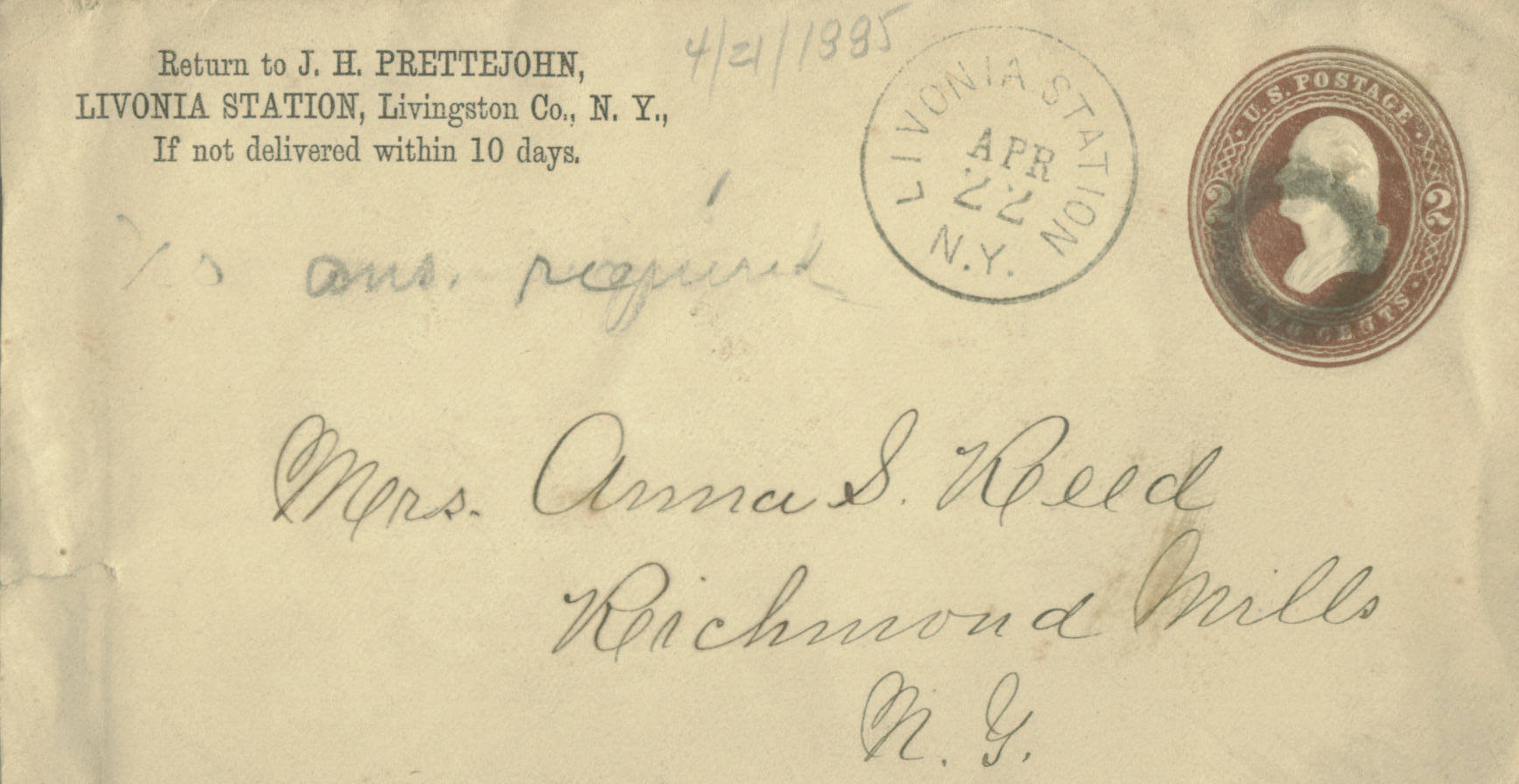This image depicts the front of an antique envelope. The upper left corner features the return address: "J.H. Prechajan, Livonia Station, Livingston County, New York," with instructions to return if not delivered within 10 days. In the top right corner, a red, circular two-cent U.S. postage stamp with a bust in the center is evident, paired with a postmark from "Livonia Station, April 22, New York." The envelope is addressed in cursive to "Mrs. Anna S. Reed, Richmond Mills, New York." Additionally, "ANS" and the date "4-21-1885" are penciled in, indicating an answer is required or requested. This piece of mail offers a rich glimpse into postal history from the late 19th century.